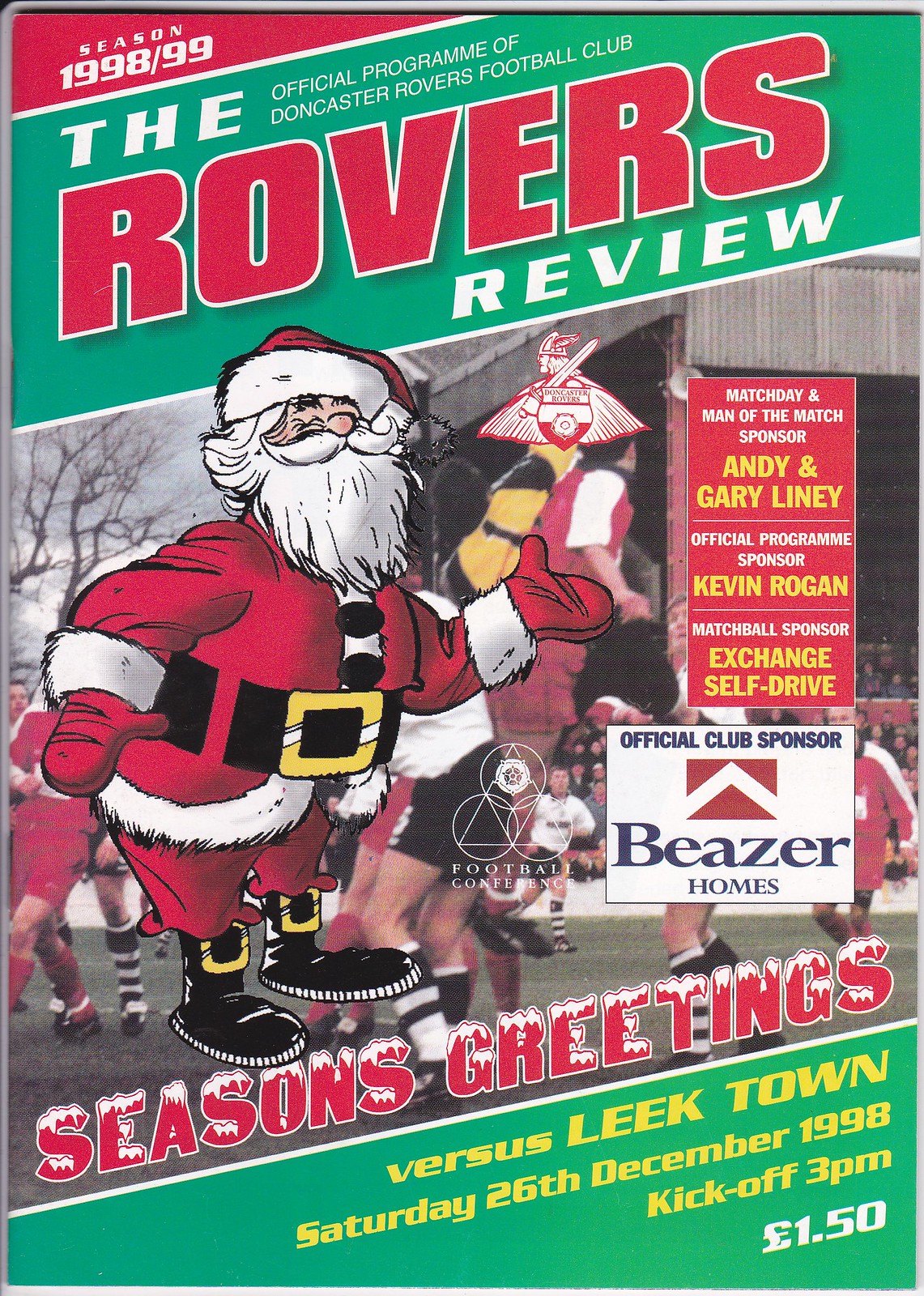This is the cover of the Doncaster Rovers Football Club's program for the Christmas season of 1998-99, prominently featuring festive green and red colors. At the top, "Season 1998-99" is displayed against a green background. The headline reads "The Rovers Review - Official Program," with a large cartoon image of Santa Claus in the center, positioned in front of football players in red kits with black boots. Along the right side, there are details about the matchday and man of the match sponsors. Beneath Santa, "Season's Greetings" is written in red letters topped with snow. Below, on a green background, the text in yellow letters announces the match against Leak Town on Saturday, 26th December 1998, with a kickoff at 3 p.m. The program is priced at £1.50.